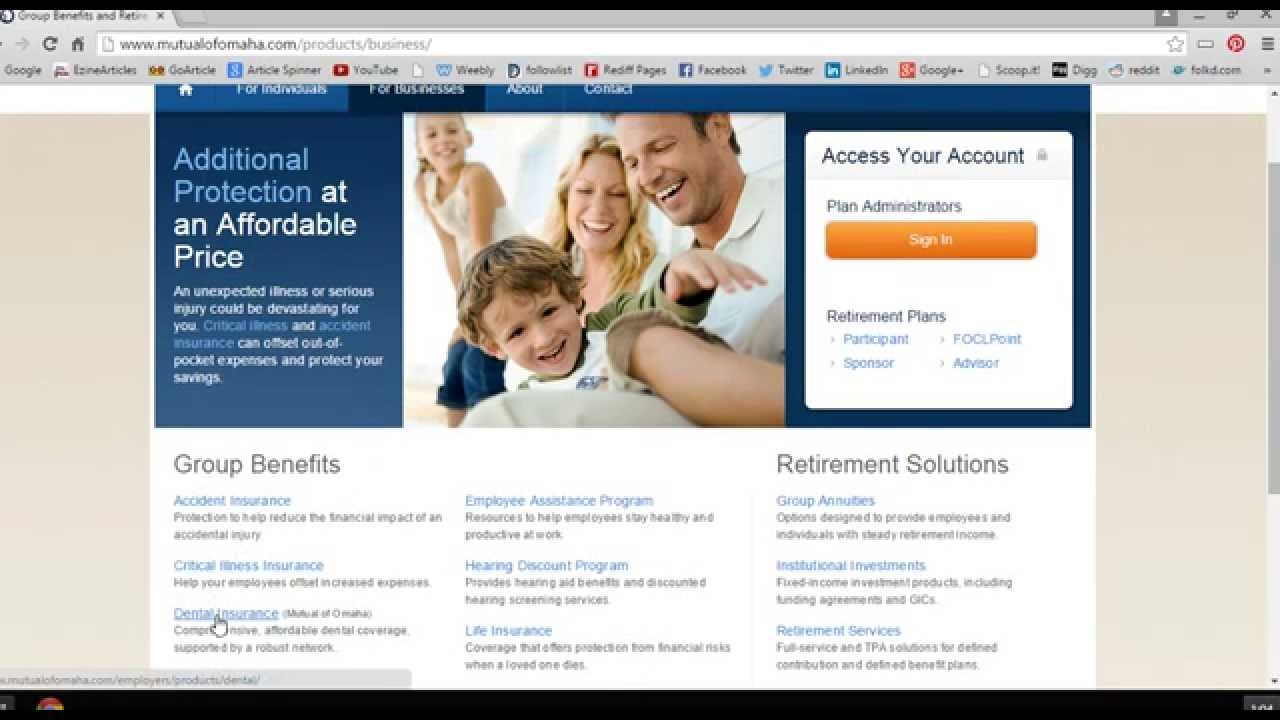This image captures the home page of a website, specifically Mutual of Omaha. It features a prominent thin black border at the top and bottom, with a gray border at the top as well. In the top left corner, there's a lighter gray pop-up tab with black text that includes options such as "Group," "Entities," and "Rating," along with a black "X" to close the tab.

The top section of the screen also shows additional elements on the right side, including a black "X," a black square, and a black minus sign. Moving to the left, there's a refresh button and a home button, followed by a long white search bar displaying "www.mutualofomaha."

Below the search bar, black words, which are somewhat blurred and hard to decipher, span across the screen. To the left of these words, various icons are visible, numbering approximately 14 or 15. In the center of the page, about two inches from both the left and right edges, a blue section stands out.

In the top left corner of this blue section, a home icon in white is visible, accompanied by four tabs with white lettering. Below these tabs is informational content about a plan. To the right of this content is an image of a family: a man on the right, a woman in the middle, a small boy in the front, and a little girl to the left in the background.

Adjacent to the family image, a pop-up tab appears, providing access to account sign-in options, retirement plans, and related information. 

Further down, there is a white section divided into three columns. The first column’s header reads "Group Benefits," followed by two columns of information. There are six clickable tabs within this section, highlighted in blue. The last column is titled "Retirement Solutions," featuring three items underneath.